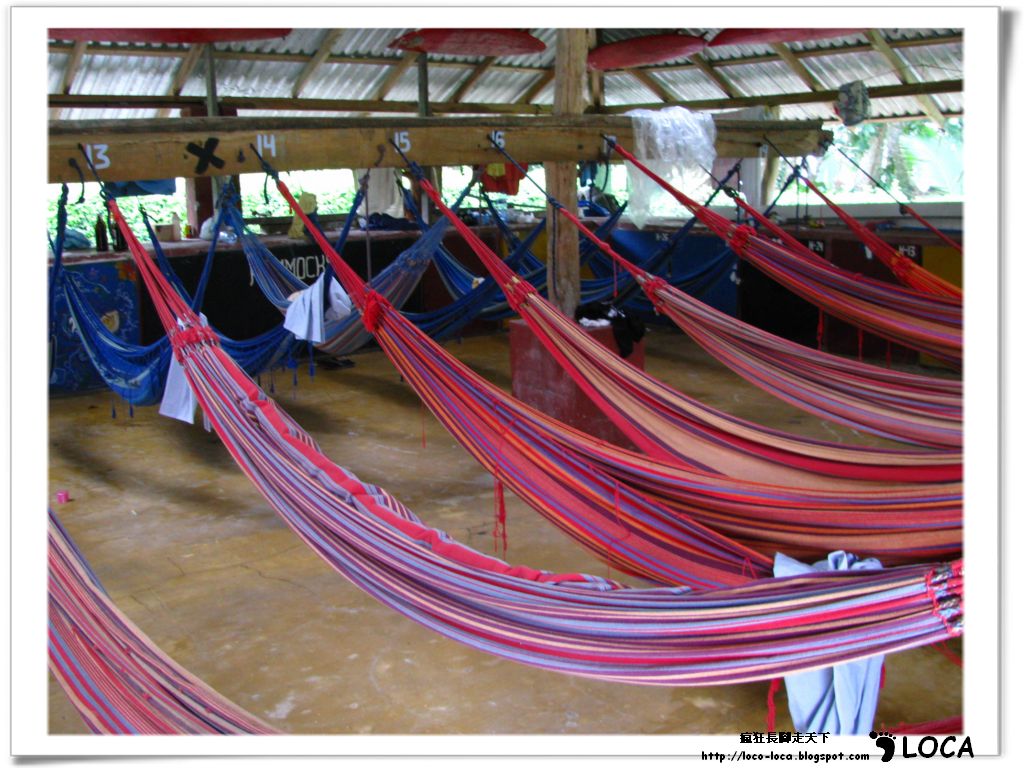The image depicts a partially open-sided building with a roof made of sealed steel sheets. Inside, there are horizontal planks running across the structure, each labeled with numbers 13 through 17. Hanging from these planks are rows of hammocks. The hammocks are predominantly red with various stripes of blue, light blue, and orange. On another parallel plank, there are additional blue hammocks. The building appears to be designed to allow light and air to flow through, creating an airy and breezy environment. Additionally, there's text in a foreign language in the bottom right corner, followed by a web address "http://www.local-local.blogspot.com". There is also a small black footprint logo next to the text. The purpose of this setup might be for renting hammocks, yet no people are visible in the hammocks within the image.